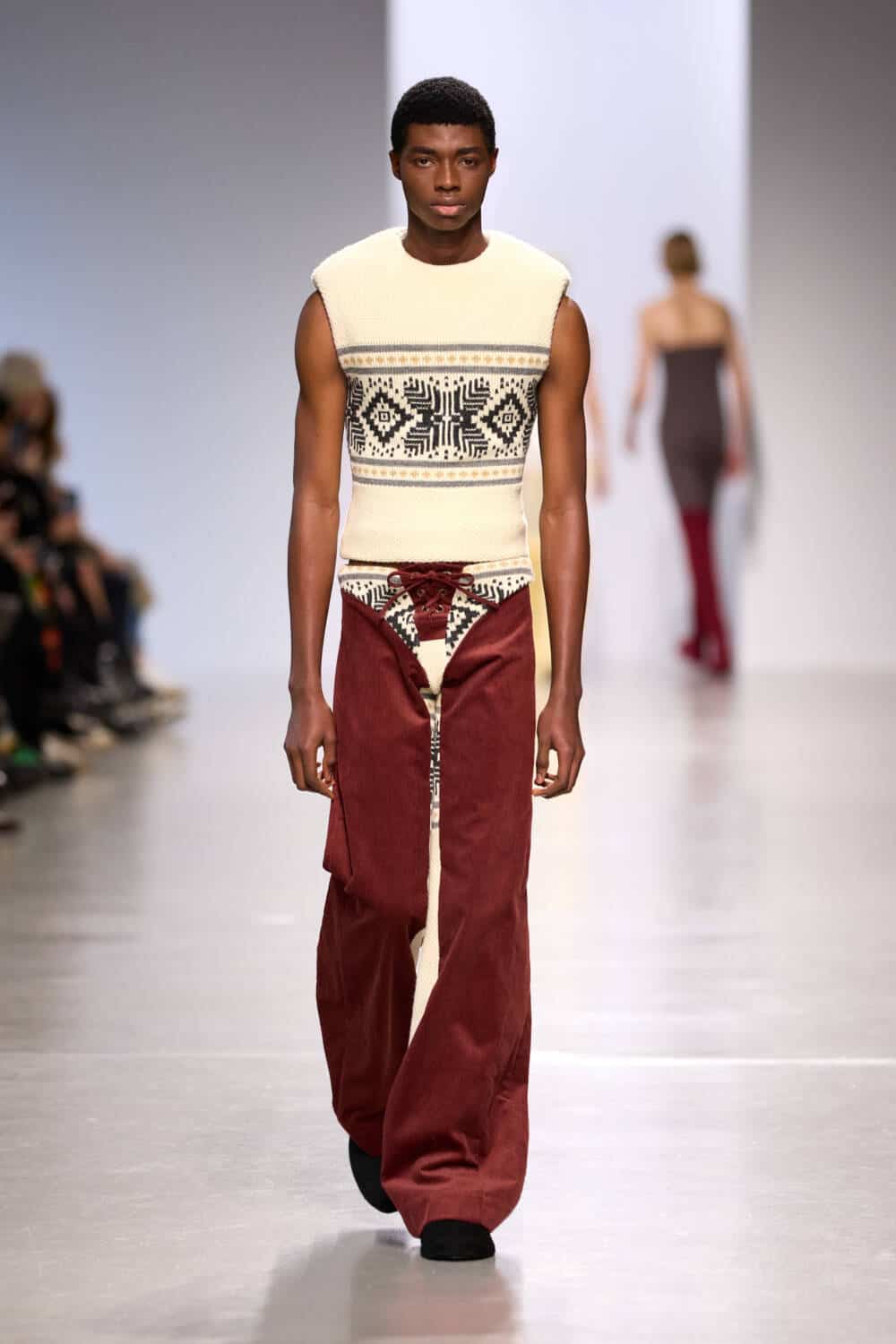In this photograph of a fashion runway, a tall African-American male model with dark skin and short black curly hair is walking towards the camera. He is wearing a sleeveless, white tank top adorned with silver and red stripes, featuring a distinctive Native American black pattern in the center. His trousers are either made of red velvet or corduroy and are designed to resemble chaps, baggy towards the bottom and tied together with strings. Over the pants, he wears an additional piece that matches the shirt in color and pattern, giving a layered, intricate appearance. Completing his look are black shoes. On the left side of the runway, the audience sits with cameras, capturing the moment, but they are out of focus, emphasizing the model's striking ensemble.